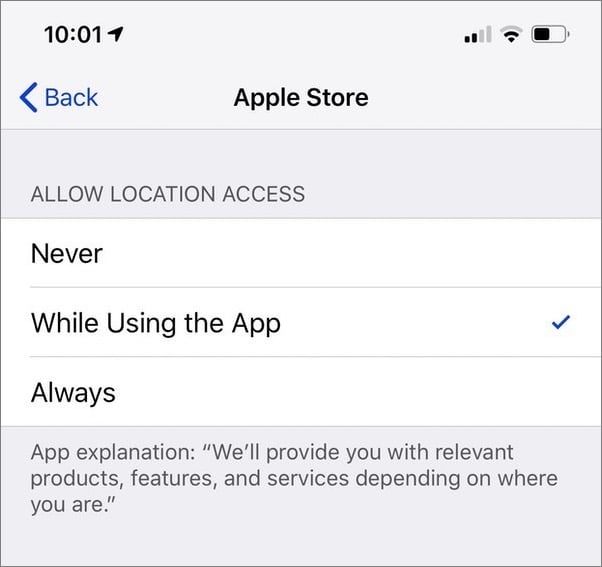This screenshot from a phone displays the interface for location access permissions within the Apple Store app:

- **Top Section:** The upper left corner shows the device time as "10:01" in black, accompanied by an upward-right pointing arrow. Adjacent to this is a set of signal bars indicating network strength, followed by an outline of the battery status.
- **Navigation Bar:** Directly below the time, a blue arrow pointing left is labeled "Back" to indicate navigation options.
- **Title:** Centrally aligned in bold black text is "Apple Store," set against a clean white background.
- **Permission Request:** Below the title, a two-inch thick gray bar presents an important request, "ALLOW LOCATION ACCESS," in all capitalized letters and darker gray font.
- **Options:** The subsequent white bar contains three options for location sharing:
  - To the left, in bold black text, "Never" is an option with a gray dividing line to its right.
  - In the center, "While Using the App" in bold black text is marked with a blue check mark.
  - Below another thin gray line, "Always" is listed in bold black.
- **Explanation Box:** At the bottom, a gray box about two to three inches thick provides further explanation in gray text. It reads: "App explanation," followed by, "will provide you with relevant products, features, and services depending on where you are."

This detailed layout offers a comprehensive understanding of the location access permissions requested by the Apple Store app.